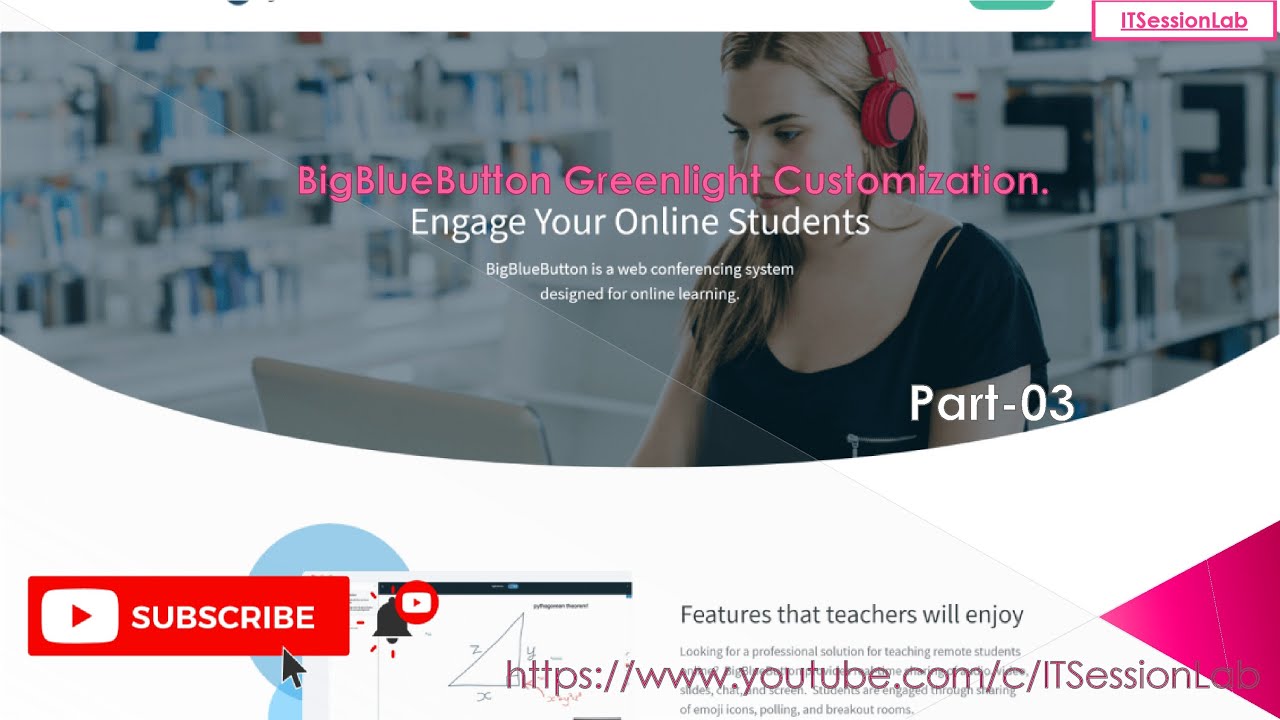This image features a woman with blonde hair sitting at a laptop, wearing red headphones. She appears to be in a store, as suggested by the various items and shelves around her. To the left side of the image, there is a display wall, and behind the woman, shelves are visible with items that look like books or thin boxes.

In the middle of the image, the text "Big Blue Button Green Light Categorization" is prominently displayed in a pinkish font that is centrally justified. Below that, in white and also center-justified, the text reads "Engage Your Online Students." In smaller, white font underneath, there is a brief description: "BigBlueButton is a web conferencing system designed for online learning."

Additionally, in the top right corner, just below the woman's left shoulder, the text "Part -03" is visible in white font.